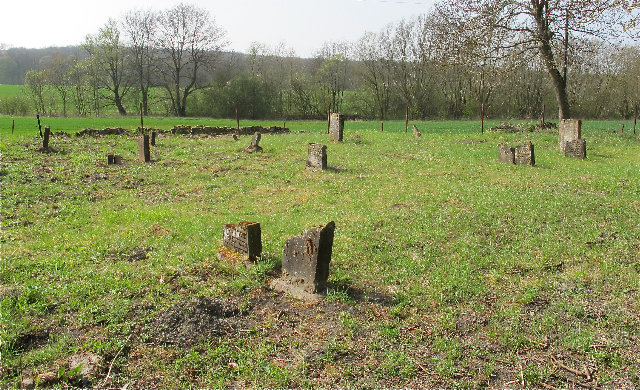The photograph captures a desolate, overgrown old cemetery set against a mixed skyline that transitions from an overexposed white on the left to a greyish-blue on the right. The foreground is dominated by patchy green grass interspersed with dirt, rocks, and twigs, enhancing the neglected atmosphere. Among the scattered tombstones, many are covered in mildew, cracked, and missing parts, with some showing jagged, broken edges. Near the forefront, two gravestones stand out; one larger but jaggedly cut off, and a smaller one still bearing some faint white inscriptions. Further back, roughly thirteen gravestones of varying sizes are randomly dispersed without any apparent order. A sparse row of trees is visible in the background, some entirely barren, allowing glimpses of the horizon beyond. The cemetery is separated from an adjacent, well-maintained field by a loosely constructed fence of stakes and wire, suggesting a divider between the neglected graves and the cared-for land next door. The overall scene conveys a sense of abandonment and decay, possibly indicating early spring given the sparse foliage on the trees and the lush green grass on the ground.